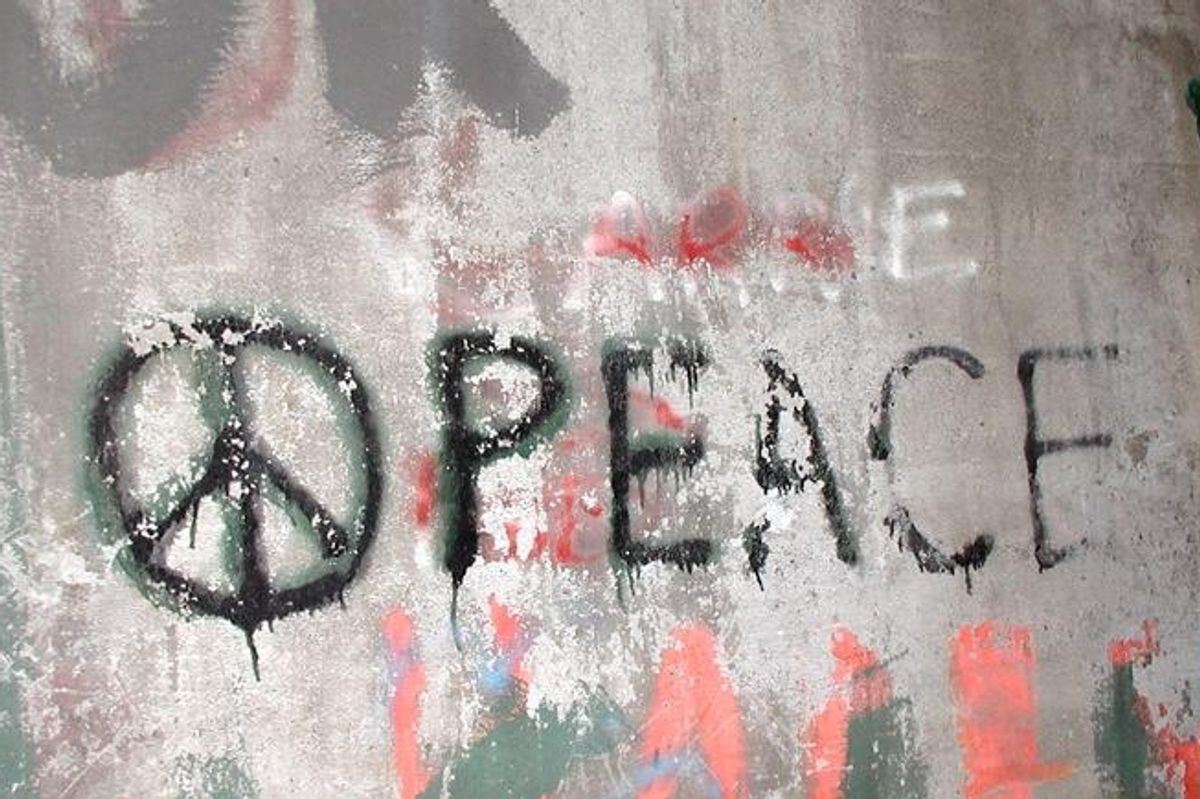The image features a concrete wall prominently marked by graffiti. The central focus is a black peace sign accompanied by the word "peace" to its right, also in black. The peace sign is backed by a gray shell and is chipping all over, with white paint stripping at the bottom. The word "peace" is partially deteriorated: the letter 'C' is missing half, and the bottom part of the 'E' is nearly gone. Surrounding the peace sign and "peace" are various tags and colors, including orange, green, and red streaks, as well as blue and mild hints of other hues. Overlapping tags in white and other colors obscure some areas. Above the primary graffiti, there appears to be text in red and white, suggesting the letters "A-R-R-N-E" or "Arnie," but it's not clearly legible. The wall is evidently a canvas for multiple layers of spray paint, contributing to its rough and weathered appearance.